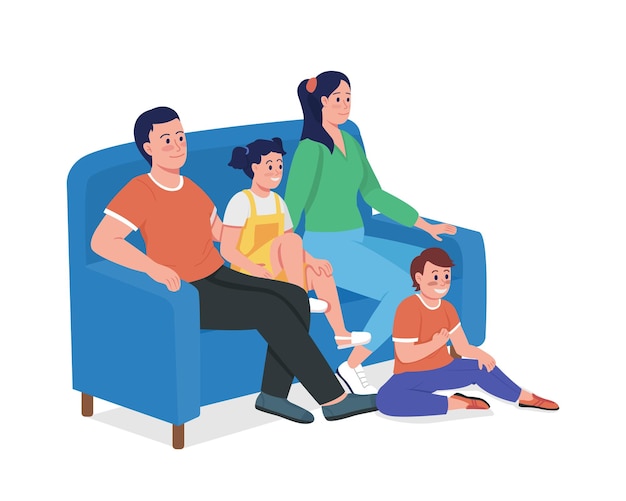The image is a simple, vector-style animated illustration of a family. The family consists of a father, mother, daughter, and son, all seated or situated around a blue couch with four wooden legs, against a white background with a shadow underneath the couch indicating a light source from above. 

The father, on the left side of the couch, is wearing an orange T-shirt, black pants, and gray shoes that might be slippers. He has dark blue hair and appears content. The mother, on the far right, has her hair in a ponytail, with either black or dark blue hair. She is wearing a green long-sleeved V-neck shirt, light blue pants, and white tennis shoes. The daughter, sitting between her parents, has dark blue hair in pigtails and is dressed in yellow overall shorts with a white T-shirt underneath. She has little espadrilles on her feet and is smiling, showing her teeth. 

The son, who looks around 12 years old, is sitting on the floor in front of the mother. He shares his father's orange T-shirt design with a white neckline and sleeve ends, and is wearing blue pants with orange shoes. He, too, is smiling, revealing his teeth. They all seem to be looking towards the right, perhaps watching television, as indicated by their expressions.